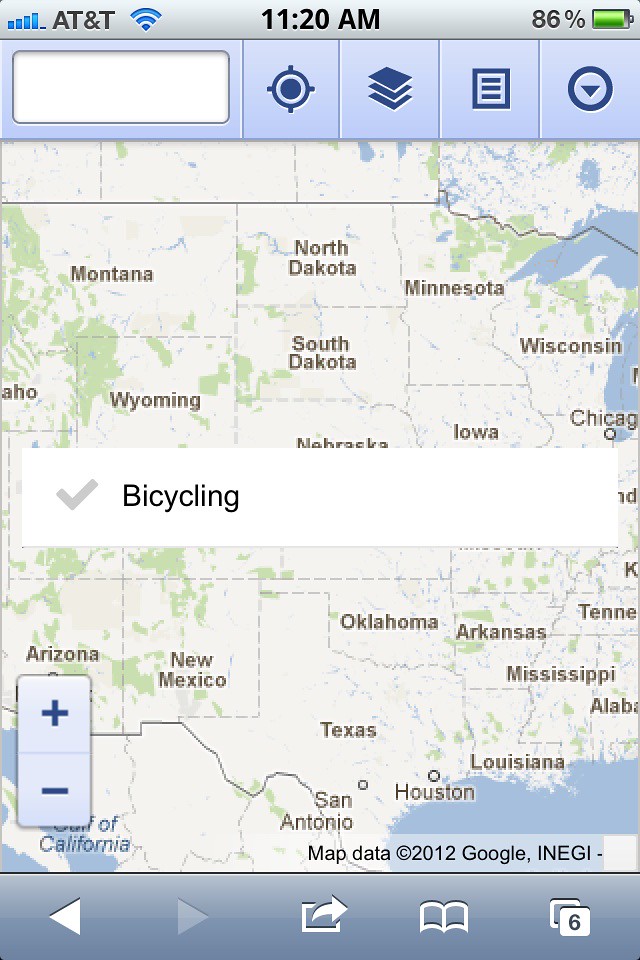This image is a vertically-oriented screenshot captured from a cell phone displaying Google Maps with specific bicycling information highlighted. The map covers the central United States, stretching from North Dakota down to Texas, without showing the East or West coasts. At the top of the screen, status indicators include the AT&T network signal, the current time (11:20), and a battery level at 86%. The interface includes a central search box, presumably used for finding bicycling routes or locations. Various controls for adding or removing map layers and bookmarking locations are visible, along with zoom in/zoom out options. At the bottom of the screenshot, map data credits are shown: "Map data ©2012 Google, INEGI."